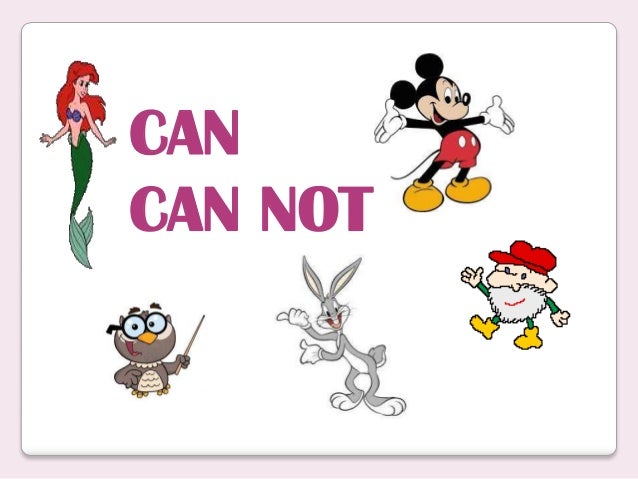The poster features a white background framed by a soft pink border. Prominently displayed at the top center is pinkish-purple text in all caps that reads "CAN" in one row and "CANNOT" in another. To the left of this text is an illustration of the Little Mermaid, depicted swimming underwater and facing right. To the right of the text, Mickey Mouse appears with open arms, smiling warmly as if launching for a hug. Below the text, an owl with glasses and a yellow beak holds a stick in front of him, positioned to the left. Adjacent to the owl, Bugs Bunny is smiling and pointing his thumb to the left, towards the owl. In the bottom right corner, there's a whimsical small character with a red hat, a gray beard, yellow shoes, and no visible body, seemingly walking and holding one arm in the air. The entire image is in full color, showcasing popular Disney characters among others, against a clean, white backdrop.